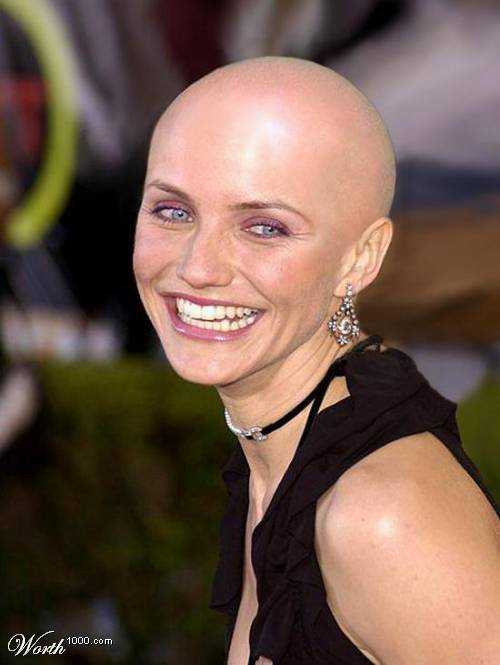This tall rectangular photograph features a close-up of a famous actress, Cameron Diaz, visible from the shoulders up. Emerging from the bottom right corner towards the top center, Diaz's completely bald head, possibly photoshopped, gleams as if freshly shaved. Her head is tilted slightly to the right, with pale, freckled skin and striking blue eyes. Displaying light brown, thin eyebrows, Cameron sports a radiant smile, revealing both her top and bottom teeth framed by bright pink lips and pink eyeshadow. One of her ears, adorned with a studded dangly earring, is visible. She is dressed in a sleeveless black ensemble, which could be described as a frilly dress, coupled with a black jeweled choker. The background is a blur of various colors including white, tan, green, yellow, red, and others, creating a dynamic, almost abstract scene. In the bottom left corner of the image, white cursive text reads "Worth," with "1000.com" positioned just above it.